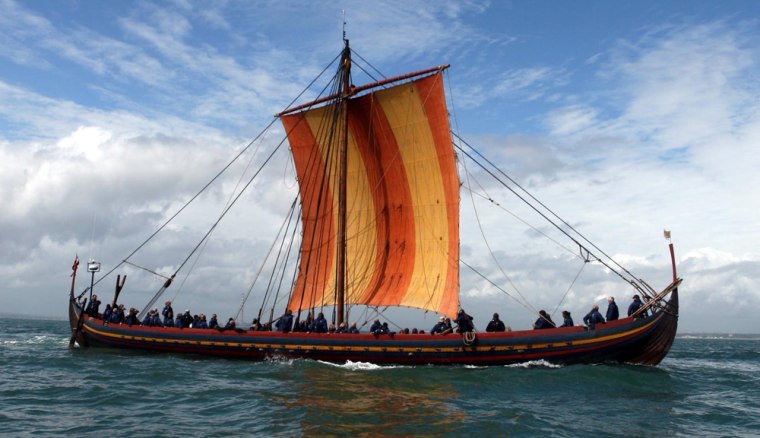This detailed photograph captures a recreated Viking boat, painted in a striking blue with a comprehensive yellow and red stripe running through its center, and a red stripe lining its railing. The boat, characterized by its single deck and pronounced upward-curving prow and stern, is visibly long and relatively low to the water. A tall, thin, brown wooden mast stands at the center, anchoring a large, rectangular sail that alternates in stripes of dark orange and yellow. Multiple black ropes and lines stretch from various sections of the boat, including the prow, bow, and central area, reaching up to different points on the mast and the horizontal yardarm that the sail hangs from. The water surrounding the vessel is calm, showcasing light ripples and a greenish hue.

The scene includes numerous individuals clad in modern long-sleeved, dark clothing, though their distant forms obscure finer details. Above, the sky presents a dramatic spectrum of weather with dark and light gray clouds giving way to clear, blue sky adorned with wispy, white clouds high above. This meticulous recreation encapsulates the essence of a Viking ship, combining historical aesthetics with modern-day elements.